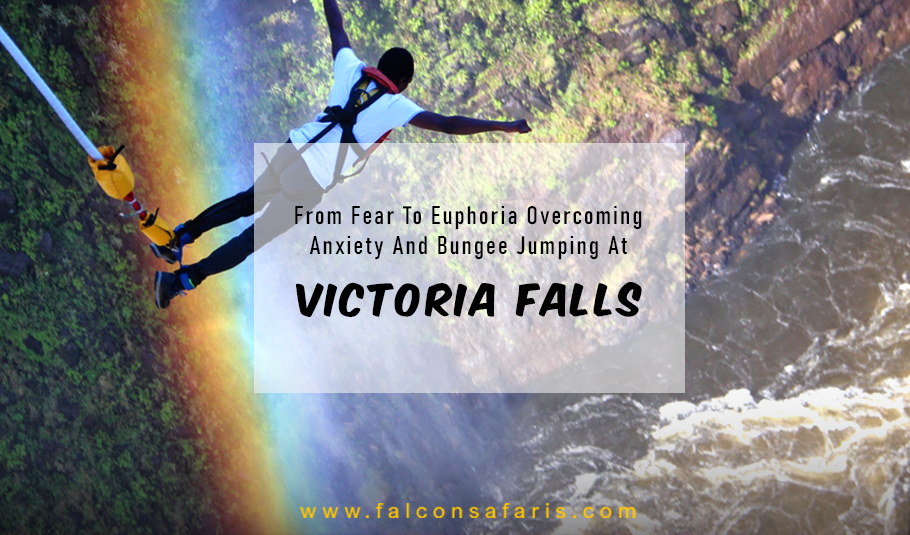This vibrant advertisement showcases the thrilling adventure of bungee jumping at Victoria Falls. Dominating the image is a dark-skinned man, outfitted in a blue shirt and red harness, plunging headfirst from a grassy cliffside towards the expansive water below. The blue bungee cord, securely fastened around his left ankle, arcs gracefully from the top left corner of the image. His vertical descent is accentuated by his outstretched arms, capturing a moment of exhilaration against the dramatic backdrop of lush, green vegetation and rugged cliffs. Beneath him, the river meanders through the canyon, reflecting a vivid rainbow with stripes of red, orange, yellow, blue, and purple, adding a dash of color and magic to the scene. Central to the image is a rectangular graphic bearing the bold message: "From Fear to Euphoria: Overcoming Anxiety and Bungee Jumping at Victoria Falls." At the bottom, the website www.falconsafaris.com invites viewers to embark on their own adrenaline-fueled journeys.